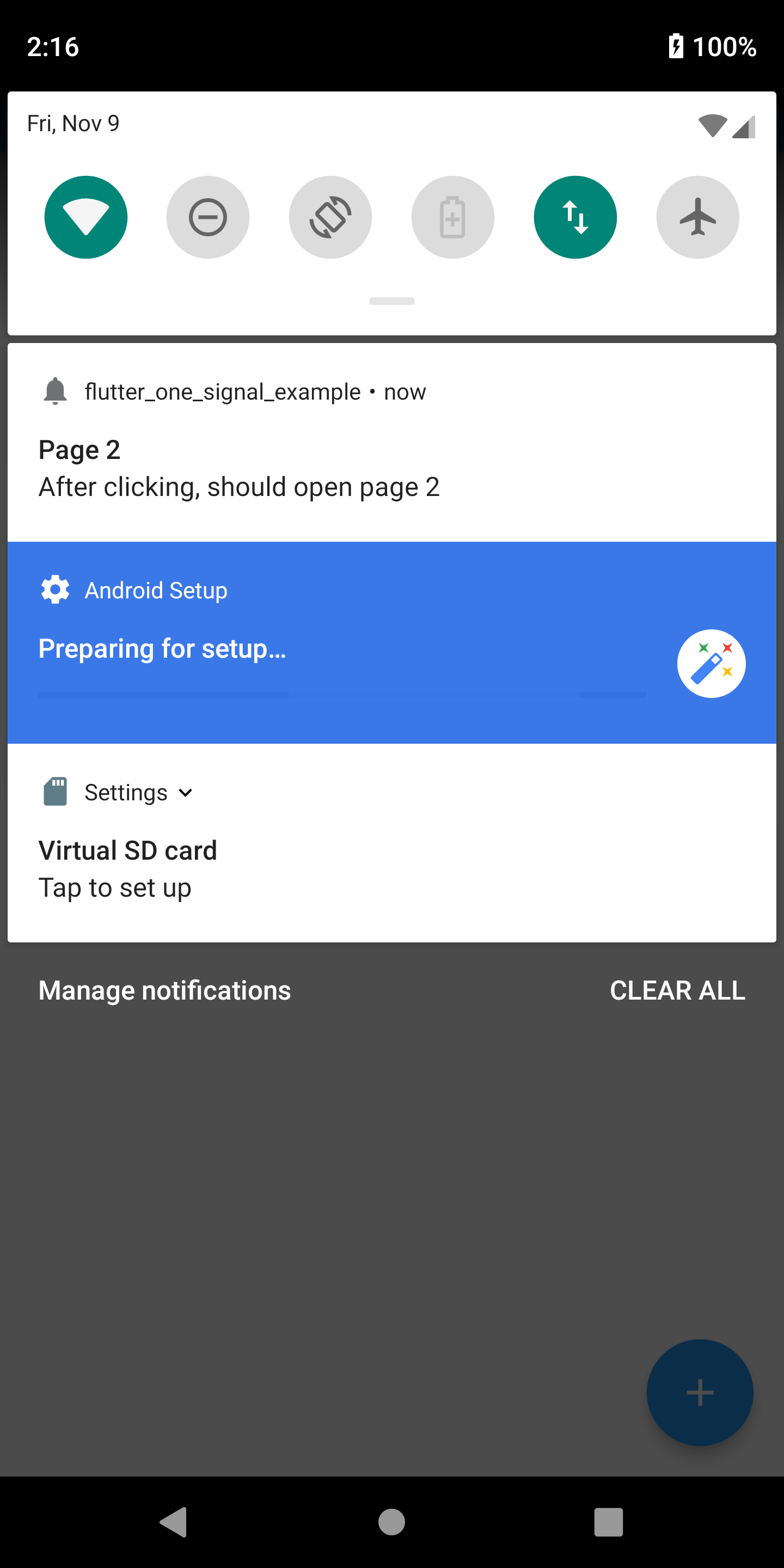This screenshot captures a mobile phone display showcasing a detailed interface. At the top, a black header features white text on the left indicating the time as "2:16," and on the right, a white battery icon with a black lightning bolt overlays it, alongside the text "100%," signifying a fully charged battery.

Below the header is a drop-down menu with a white background. In the top left corner, dark gray text reads "Friday, November 9th (NOV)." The menu includes six icons: the first, a Wi-Fi symbol in white on a teal circular background, symbolizing Wi-Fi connectivity. Adjacent to it are three icons with light gray backgrounds, the first two featuring dark gray icons. Notably, one of these icons depicts a battery with a plus symbol in the center. Another teal icon displays two white arrows, one pointing up and one pointing down, likely indicating data transfer. The following icon is a dark gray plane on a light gray circular background, representing airplane mode. 

Centrally positioned at the bottom of this section, a thin, light gray pill-shaped bar rests above a thin black line, segregating the drop-down menu from three notifications below.

The first notification, with a white background, starts with a dark gray bell icon in the top left, followed by dark gray text stating "Flutter_1_signal_example." A small dot separates this from the word "Now." Directly below, black text left-justified reads "Page 2," with slightly smaller text beneath stating, "After clicking should open Page 2."

The middle notification stands out with a blue background and contains white text and icons. Lastly, the third notification also on a white background is labeled "Settings," mimicking the style of the first notification.

Below these, on the left side, bold white text hovers over the background saying "Manage Notifications," while on the right, in all capital letters, white text states "CLEAR ALL."